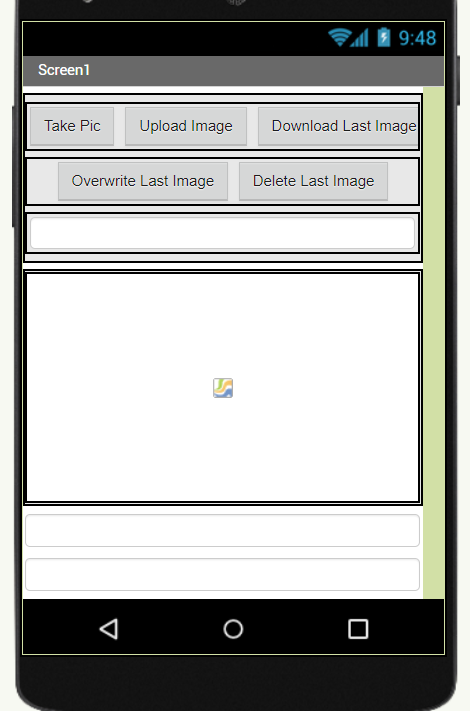A screenshot displays a window with a black background and a top black header showing phone signal, Wi-Fi signal, full battery, and a time stamp of 9:48 in the top right corner. The browser window features a very light lime green outline. Directly below the header, there is a narrow grey stripe labeled "Screen 1" on the left side. Beneath this stripe, a white box contains two rows of buttons. The first row from left to right includes buttons labeled "Take Pic," "Upload Image," and "Download Last Image." The second row contains "Overwrite Last Image" and "Delete Last Image." In the center of the window is a white section with a square in the middle, showcasing green, orange, and blue swirls, indicating a likely unsuccessful image load.